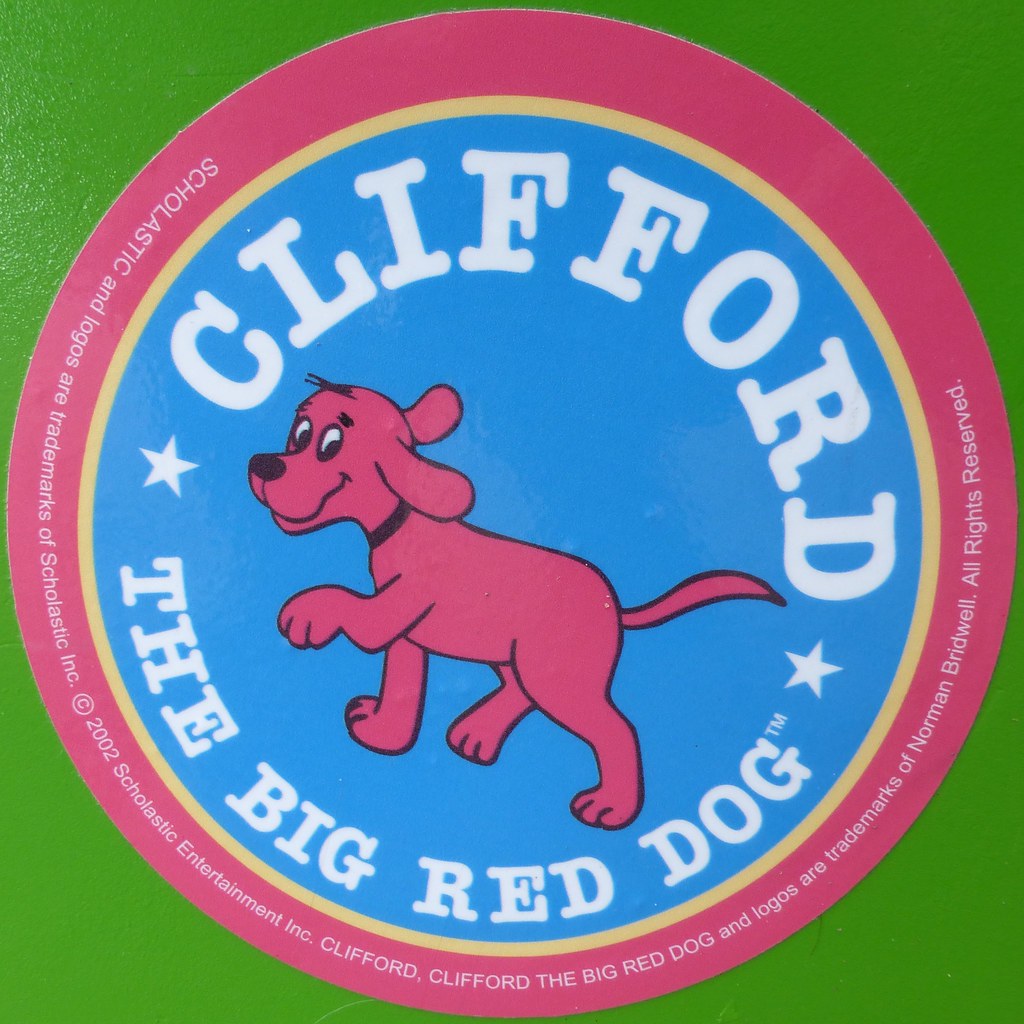In the image, a vibrant green background frames a pink circular border. Within this pink circle, there is text that reads: "Scholastic and logos are trademarks of Scholastic Incorporated, Copyright 2002, Scholastic Entertainment Incorporated. Clifford, Clifford The Big Red Dog, and logos are trademarks of Norman Bridwell. All Rights Reserved."

Inside the pink circle, a smaller yellow circle encloses yet another inner blue circle. Positioned at the top of the blue circle, the word "Clifford" is written in white, forming a semi-circle. Below the text, there is a playful illustration of a red dog. This cartoon dog has a black nose and eyes that are looking towards the left. Its tail is up in the air, and one of its paws is lifted. The dog also sports a black collar around its neck.

Flanking the dog illustration, there are stars on either side. Beneath the dog, in another white semi-circle, the text reads: "The Big Red Dog," followed by the abbreviation "T.M." This charming canine character is clearly identified as cartoonish in style, embodying the beloved depiction of Clifford, The Big Red Dog.